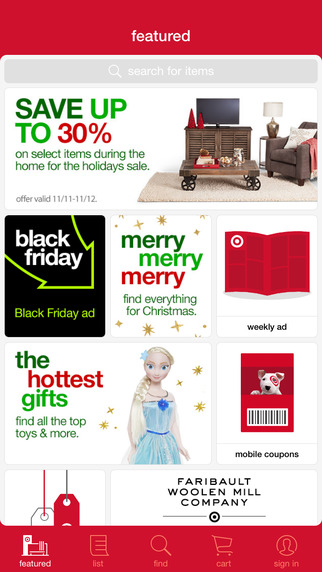The image displays a screenshot of the Target app interface, emphasizing its festive holiday promotions. At the top of the image, the word "Featured" is prominently displayed in red against a white background. Below this is a white search bar on a gray background, with the prompt "Search for Items."

The main promotional banner showcases a "Home for the Holiday Sale," offering up to 30% off on select items, valid from November 11th to November 12th. The sale's vibrant red and green Christmas-themed color scheme sets a festive tone.

On the right side of the promotion, part of a cozy living room is visible. It features a TV atop a cabinet, an unusual coffee table with wheels, a brown chair, and a simple silver and white lamp on a silver end table, all set on a white carpet.

The app interface is divided into several sections:

1. A "Black Friday" section with a green-neon arrow labeled "Black Friday ad."
2. A section labeled, "Merry, Merry, Merry Find Everything for Christmas," directing users to Christmas-related items.
3. A "Weekly Ad" section reminiscent of traditional Target advertisements.
4. "The Hottest Gifts" section featuring popular toys, including what appears to be an Elsa doll from Disney's Frozen.
5. "Mobile Coupons" section, with an image of the Target dog and a barcode.

Further down, partially cut off, are visible price tags and a reference to "Faribault One Mill Company." At the bottom navigation bar of the app, the sections "Featured" (highlighted), "List," "Find," "Cart," and "Sign In" are visible, indicating that the user is not currently signed in. 

Overall, the screenshot reflects Target's user-friendly app design, packed with holiday deals and user-centric navigation features.